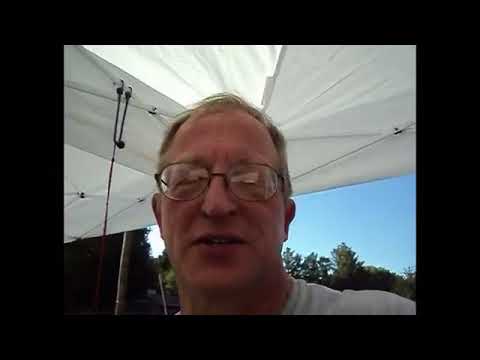The image portrays an older man, possibly in his fifties, wearing wire-framed glasses that reflect light. His hair is thinning and appears to be a mix of brown and silver. He is dressed in a light gray or white t-shirt. The man’s mouth is slightly open, suggesting he is mid-sentence or perhaps just smiling faintly, with eyes partially closed. Positioned under a white tent-like canopy, the scene suggests an outdoor setting, possibly at an event like a golf tournament. The background features a light blue sky and a canopy of green trees, indicating a pleasant, sunny day. The photo has a grainy quality with a black border encompassing it, implying it may have been taken from a video or with an older camera.